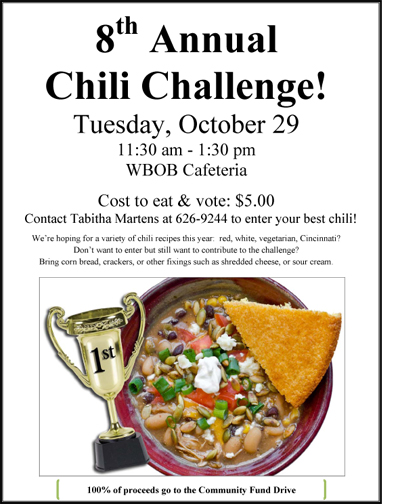The image is a white poster-style advertisement with a black border featuring promotional details for the 8th Annual Chili Challenge. The event is scheduled for Tuesday, October 29th, from 11:30 a.m. to 1:30 p.m. at the WBOB Cafeteria, which might be associated with a radio station. In bold black letters, it announces that the cost to eat and vote is $5, with all proceeds benefiting the community fund drive. Participants are encouraged to contact Tabitha Martins at 626-9244 to enter their best chili recipes. The flyer calls for a variety of chili types, including red, white, vegetarian, and Cincinnati styles, and invites contributions of side dishes such as cornbread, crackers, shredded cheese, or sour cream for those not entering the chili competition. At the bottom of the flyer, there is an image of a first-place trophy next to a vibrant bowl of chili garnished with beans, sour cream, and a slice of cornbread, reminiscent of a colorful salsa.